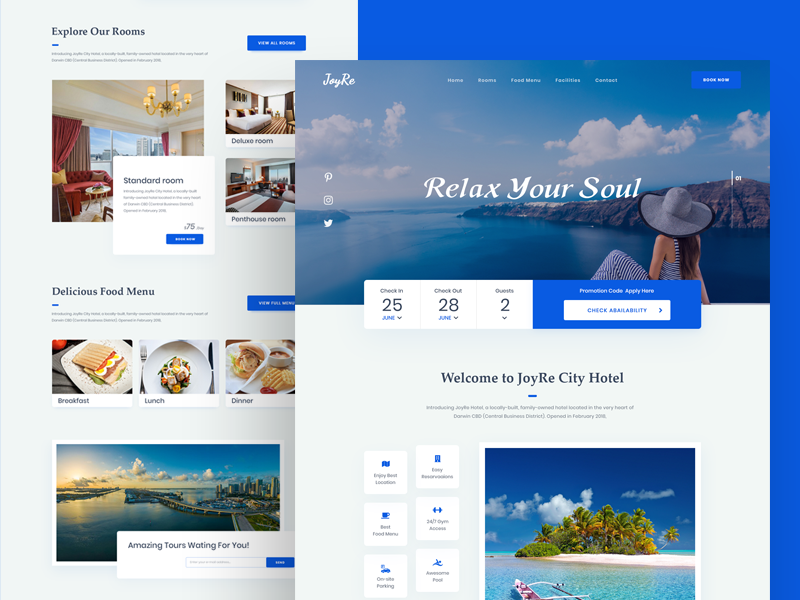Here's a detailed and cleaned-up descriptive caption for the image:

---

The hotel booking website showcases a visually appealing layout with an aesthetic that blends various shades of bright and medium cobalt blue, which seamlessly integrates with the sky visible in some of the photos. The background is predominantly a pale blue, split evenly from left to right, with a series of photos overlaid.

In the upper left corner, the heading reads "Explore Our Rooms" with a darker blue button labeled "View All Rooms." Below this heading, there are three photos: one larger image flanked by two smaller thumbnails on its right side. A white text box in the foreground highlights the "Standard Room."

To the right of this setup, occupying the cobalt blue area, another graphic box is partly superimposed. It features an Oceanside photo with the heading "Relax Your Soul." This appears to be the primary booking interface, displaying fields for "Dates," "Check In" (25th), "Check Out" (28th), "Guests" (2), and the button "Check Availability."

Beneath this section, against a white background, the welcome message "Welcome to Joyre City Hotel" is prominently displayed. To the left, six small buttons outline various amenities. To the lower right corner, there's a thumbnail of an inviting tropical scene with an ocean view and a greenery-clad island under a blue sky.

In the lower left corner, under the heading "Delicious Food Menu," there are thumbnails showcasing breakfast, lunch, and dinner options. Just below this, another photo features the text "Amazing Tours Waiting for You," depicting a picturesque city by the ocean, enhancing the allure and inviting nature of the destination.